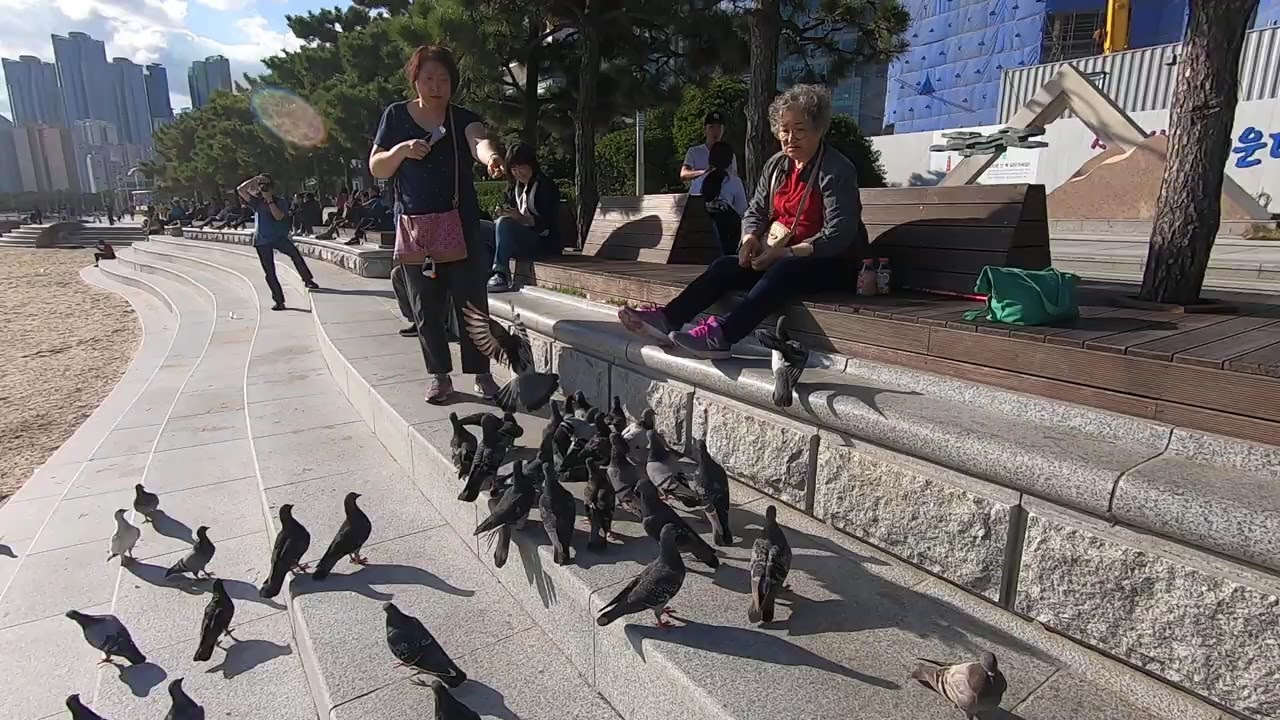In a vibrant color photograph capturing a sunny day in a park, two older Asian women are engaged in feeding a flock of around 40-50 pigeons on a long row of stone steps. The woman on the left, possibly in her 50s, is standing with her arm extended, likely offering food to the birds. She has dark, short hair and is dressed in a blue shirt, black pants, and a pink purse slung over her shoulder. To her right, seated two steps above, is an older woman, perhaps in her 60s or 70s, with gray hair and glasses, wearing a red shirt, a blue jacket, and jeans. Surrounding them is a lively scene of pigeons, predominantly grey and white, clustering around the women in anticipation. 

In the background, several people are scattered on the steps, one of whom appears to be photographing the scene. The park is bordered by a row of pine trees, a blue and white building with an artistic triangular sculpture, and noticeable construction activity. To the left, a sandy area suggests proximity to a beach. Towering above are tall skyscrapers under a clear blue sky dotted with white clouds, completing the bustling yet serene urban park setting.